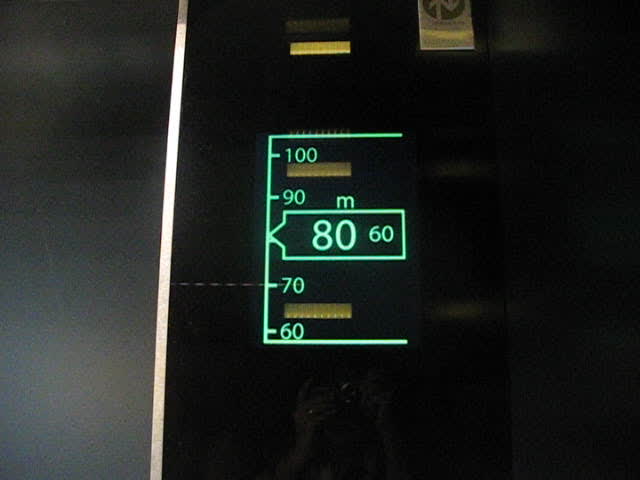The image depicts a screen with a predominantly black background that features a subtle gradient, making it lighter on the left side. A vertical white line extends downward from a point slightly off-center at the top of the screen, tapering from a wider top to a narrower base.

On the right side of the white line is a graphic resembling the letter "E" without its middle line. At the top of this "E"-like icon, there are numerical labels "100" and "90". Around the position where "80" should be, the graphic incorporates an icon resembling a battery shape—it tapers to a point, dips down, then rises to form a rectangle. This area prominently displays "80" in large print with "60" in smaller print beneath it. Further down, the numbers "70" and "60" are shown, with a dash extending from the "E"-like structure towards the white line at the level of "70".

Above the "E"-shaped figure, a yellow tab is visible. The section of the "E" that includes the battery-like shape is illuminated in green, adding a distinct color element to the image.